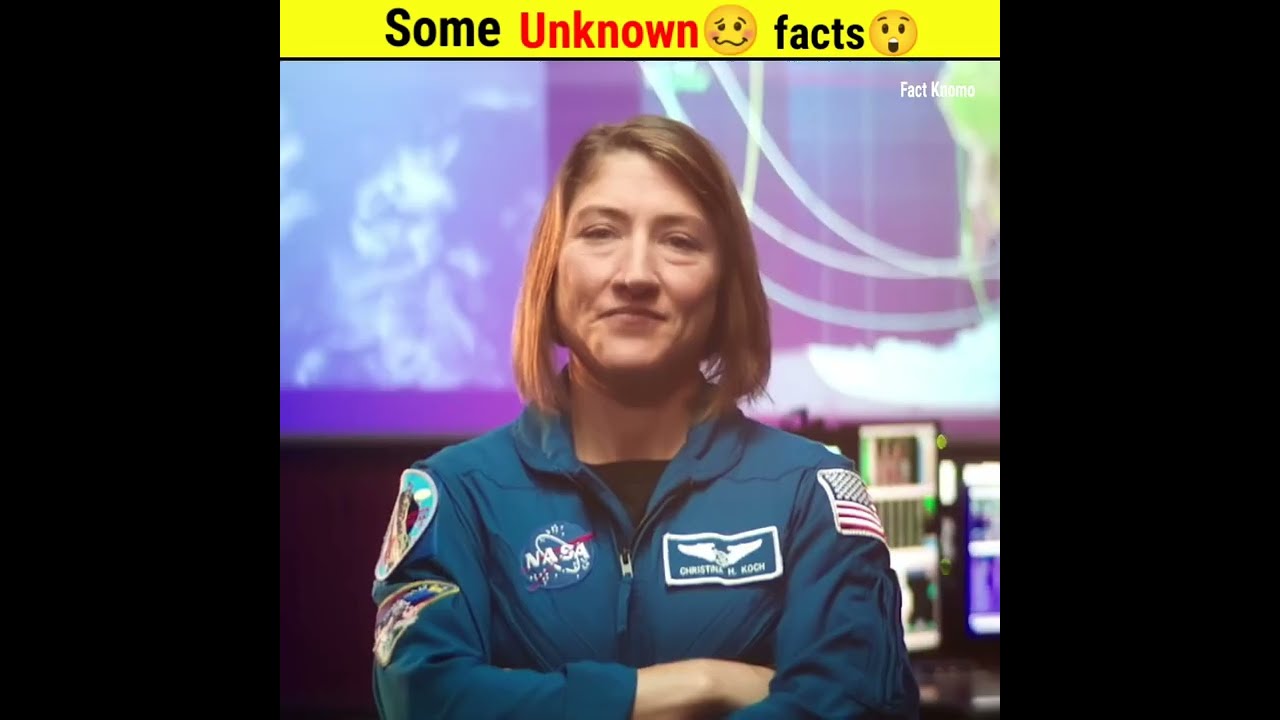This image features a Caucasian woman, likely an astronaut or NASA personnel, standing prominently in a NASA control room. She is the focal point of the photograph, which shows her smiling subtly with her lips closed. Her light brown, chin-length hair is parted on the right, and she displays a few facial lines, suggesting she is older. She is dressed in a blue NASA zip-up jacket with a NASA logo on the right breast, possibly an eagle emblem with wings and a white rectangular name patch reading "Christina Koch." Additionally, her uniform features an American flag patch on the left shoulder and several other patches on the right. Underneath her jacket, she wears a black t-shirt. The background of the image is blurred but reveals large display screens showcasing orbits or space-related visuals, possibly including planetary objects, space shuttles, or satellites. There are also monitors and a desk visible behind her. The top of the image contains a thin yellow header with a light gray border; printed within the header are the words "Some Unknown Facts" in black and red, accompanied by a couple of emoticons. The photo itself has black borders on the left and right side, adding to its framed appearance.